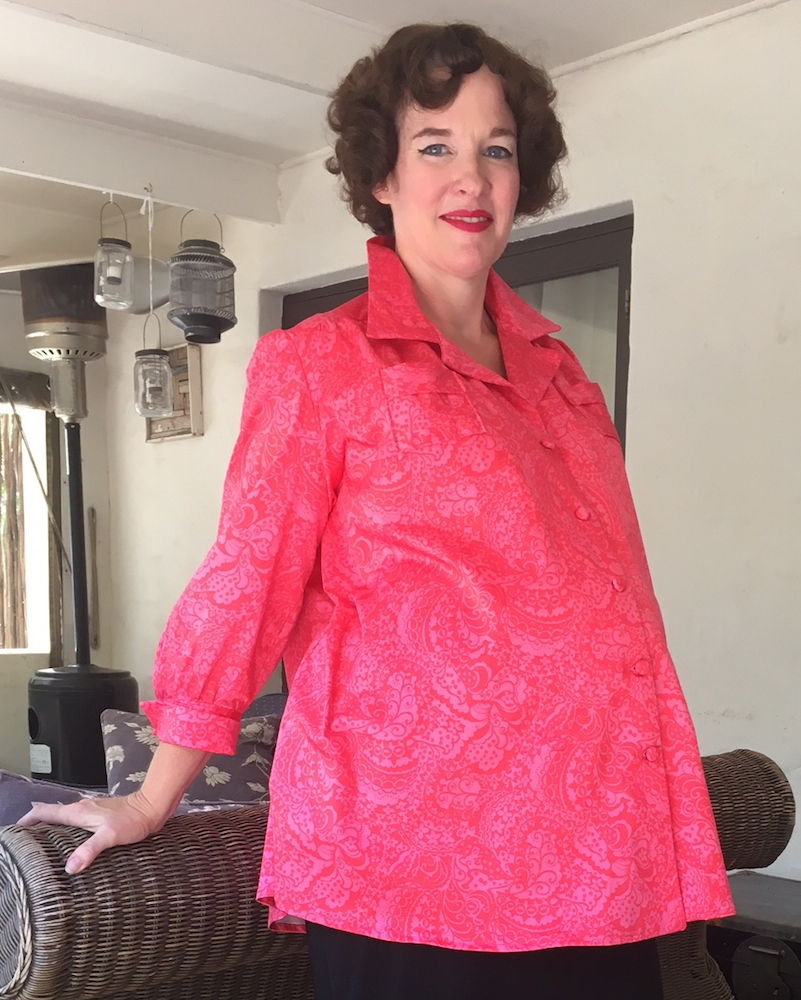In a warmly lit indoor setting, a white woman in her thirties is the focal point of this elegant photograph. She is dressed in a vibrant red floral maternity top with a collar and long sleeves, indicating her pregnant state. Her short, neatly styled brown hair frames her face, highlighting her striking blue eyes and red lipstick. The woman's gentle smile is turned towards the camera as she leans back against the wicker arm of a sofa, her right hand resting on its edge for support.

The background reveals a cozy, slightly rustic ambiance. A white wall with a passageway gives a glimpse into another room, while overhead, three distinct hanging items—a couple of mason jars and a vintage-style lantern with a candle inside—lend a touch of charm to the scene. To the left, an outdoor propane heater with its tall, cylindrical base and prominent heating element stands near a window, further contributing to the warm light that fills the room. The overall atmosphere captures a tranquil and intimate moment, with the woman's content expression perfectly embodying the serene environment.